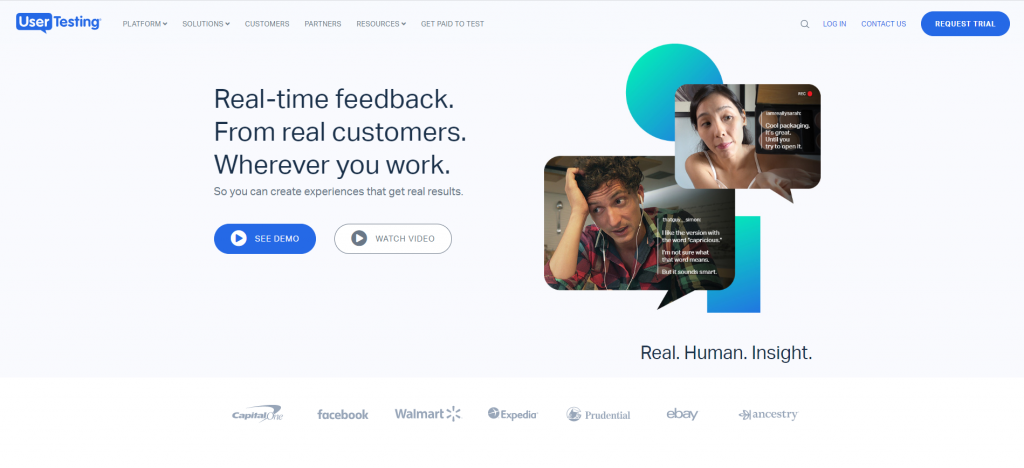On a clean, white background, the UserTesting website’s sign-up page prominently features their logo in blue at the upper left, labeled "UserTesting." Following the logo are menu options: "Platform" (with a dropdown), "Solutions" (with a dropdown), "Customers," "Partners," "Resources" (with a dropdown), and "Get Paid to Test." To the right of these options, users can see icons and links for a search (magnifying glass icon), "Log In," "Contact Us," and a "Request Trial" button in bold blue with white text.

Centrally displayed is the core message: “Real-time feedback.” followed by “From real customers.” and “Wherever you work.” Below these, in smaller font, the text reads: “So you can create experiences that get real results.” 

Beneath this message, two call-to-action buttons are visible. The first button, labeled “See a Demo,” is blue with white text. The second button, labeled “Watch a Video,” features white text and a gray outline on a black background.

To the right of the central text, there is an image of two people engaging with the platform: a woman who comments, “Cool packaging. It’s great until you try it again.” and a man who adds, “I like the version with the words something.” Despite the poor resolution, it is evident that the website emphasizes obtaining insights from real humans.